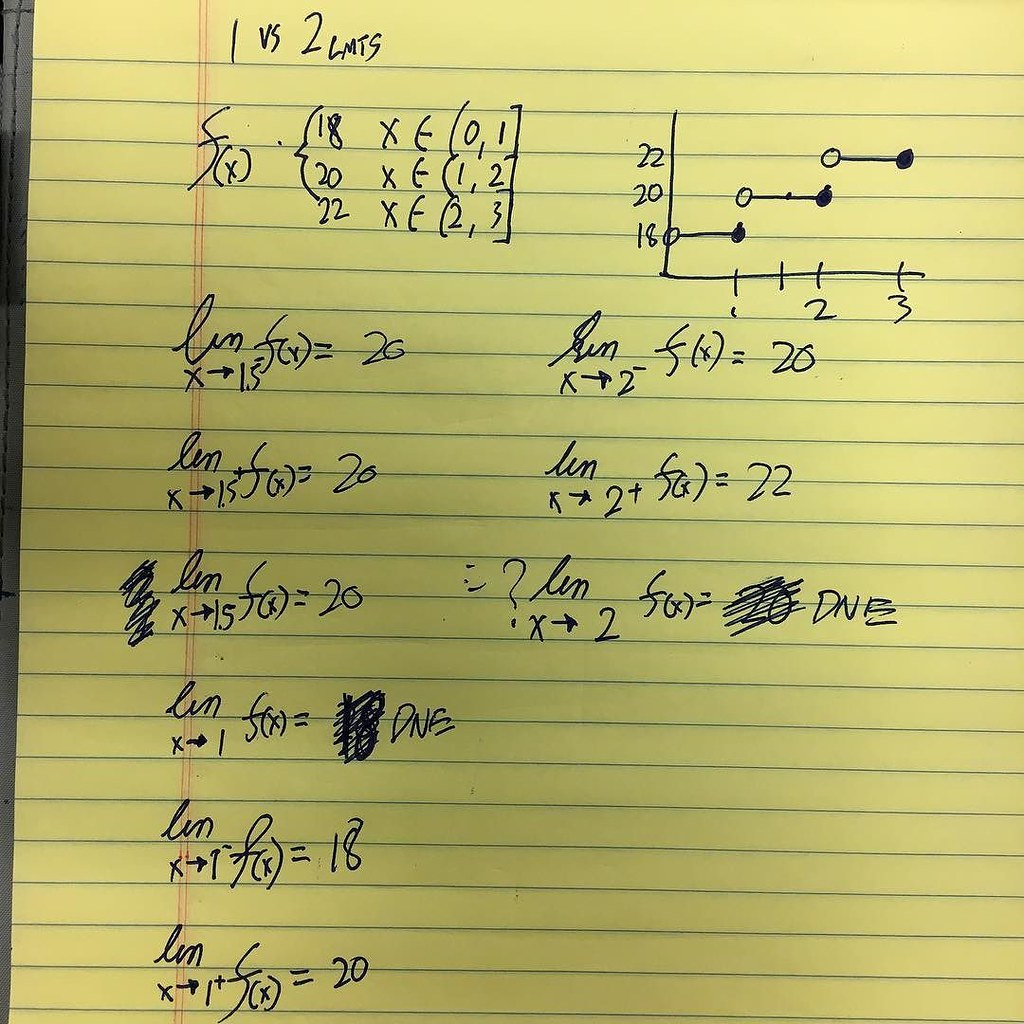This is an image of a yellow legal pad prominently featuring horizontal blue lines and a double vertical red line approximately two inches from the left margin. At the very top in blue ink, the pad is labeled "one versus two." Below this heading, the formula "F times" and bracketed numbers (18), followed by what appears to be the letter "E," are repeated down the page. 

The content consists of various mathematical problems: on the left side, "LEN" precedes "15 + FX = 20," which is listed multiple times. Another common formula seen is "X times 1 = 18," similar to the previous one involving "LEN" or "LIN" — it sometimes appears as an "E" or "I."

In the top right corner, the numbers 22, 20, and 18 are vertically aligned, separated by a vertical line. Above this line are the numbers 1, 2, and 3, each followed by an open circle and a closed, colored-in circle, with a line connecting each number to the respective circles.